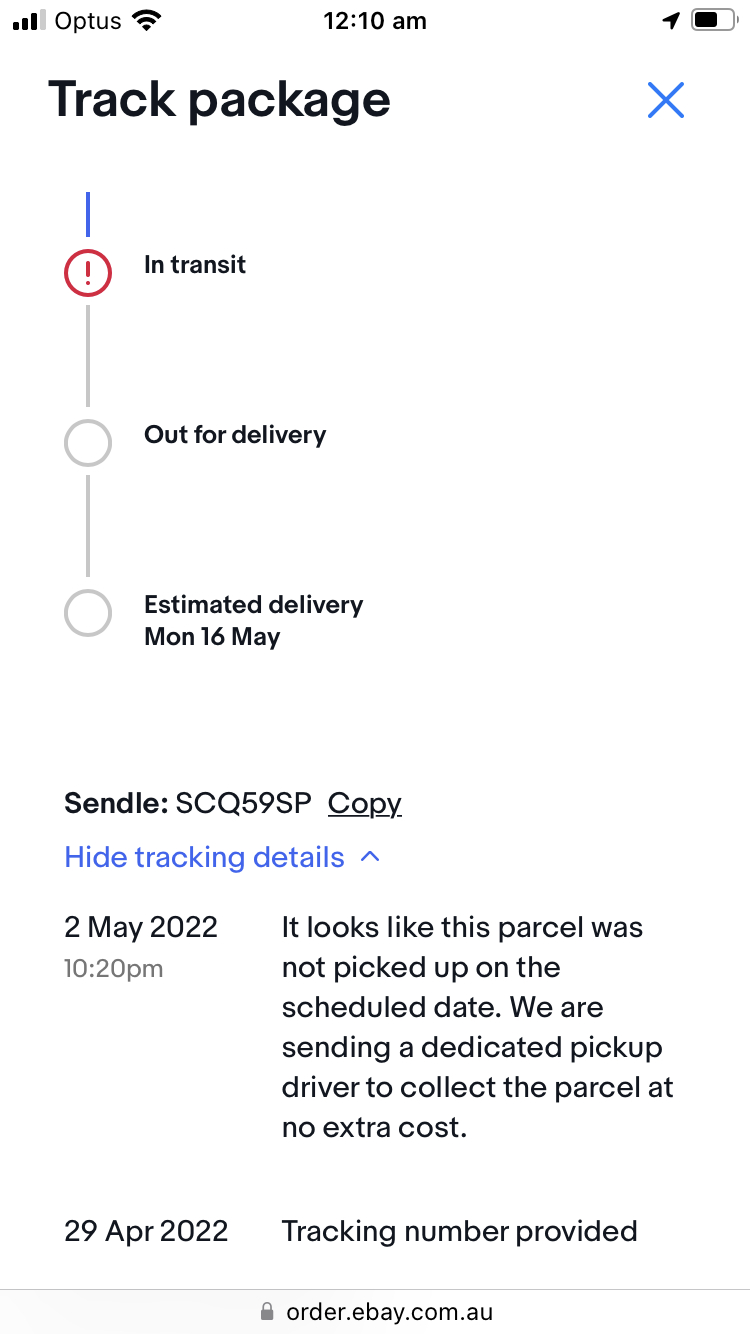This screenshot is taken from an eBay package tracking page. At the very top, bold black text prominently displays "Track Package," accompanied by a blue "X" icon to the right. Below this, a timeline composed of vertical lines and circles runs down the left side of the page, indicating the shipping progress. 

The first circle is red with an exclamation point inside it and is labeled "In Transit." The middle circle is grayed out with the label "Out for Delivery" to its right. The bottom circle is also gray and notes the "Estimated Delivery: Monday, 16th of May." 

Further down, it shows the term "CINDL" followed by a tracking code, which can be copied by clicking the adjacent "Copy" text. There's an option to "Hide Tracking Details" in blue text below this section. 

Going into more detail, an entry listed on "2 May 2022, 10:20 PM" states that, "This parcel was not picked up on the scheduled date. We are sending a dedicated pickup driver to collect the parcel at no extra cost." Another entry, dated "29 April 2022," mentions that the tracking number was provided at that time. The screenshot's bottom contains a gray banner displaying "order.ebay.com.au."